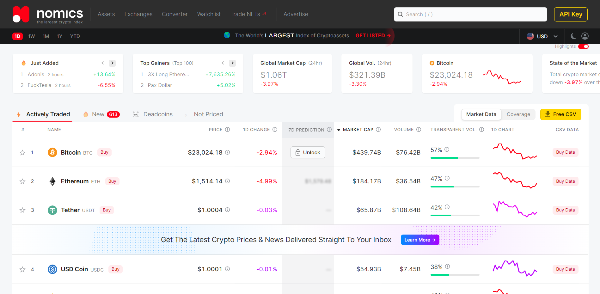On the Gnomonics website, the screen appears to be minimized, making the text difficult to read. The top part of the screen features two black bars that stretch across the width. The uppermost bar is gray and displays the Gnomonics logo and six categories in white text. Adjacent to these categories, there's a search bar and a yellow-outlined box labeled "API key."

Beneath these elements is a smaller black bar featuring five menu options, with the letter "D" highlighted in a red box. Moving to the center of the top bar, some additional text is visible. On the far right, icons for an American flag (indicating USD), an account, and a half-moon symbol are displayed.

Below these navigational elements, the main content focuses on stock market trends. Data is organized into rows and columns, showcasing various cryptocurrencies. Notably, the Bitcoin section indicates a net profit, which is displayed in red if negative and black if positive. Each cryptocurrency entry is accompanied by a line graph illustrating its trend, either upward or downward. Overall, the page displays information for a total of four different cryptocurrencies.